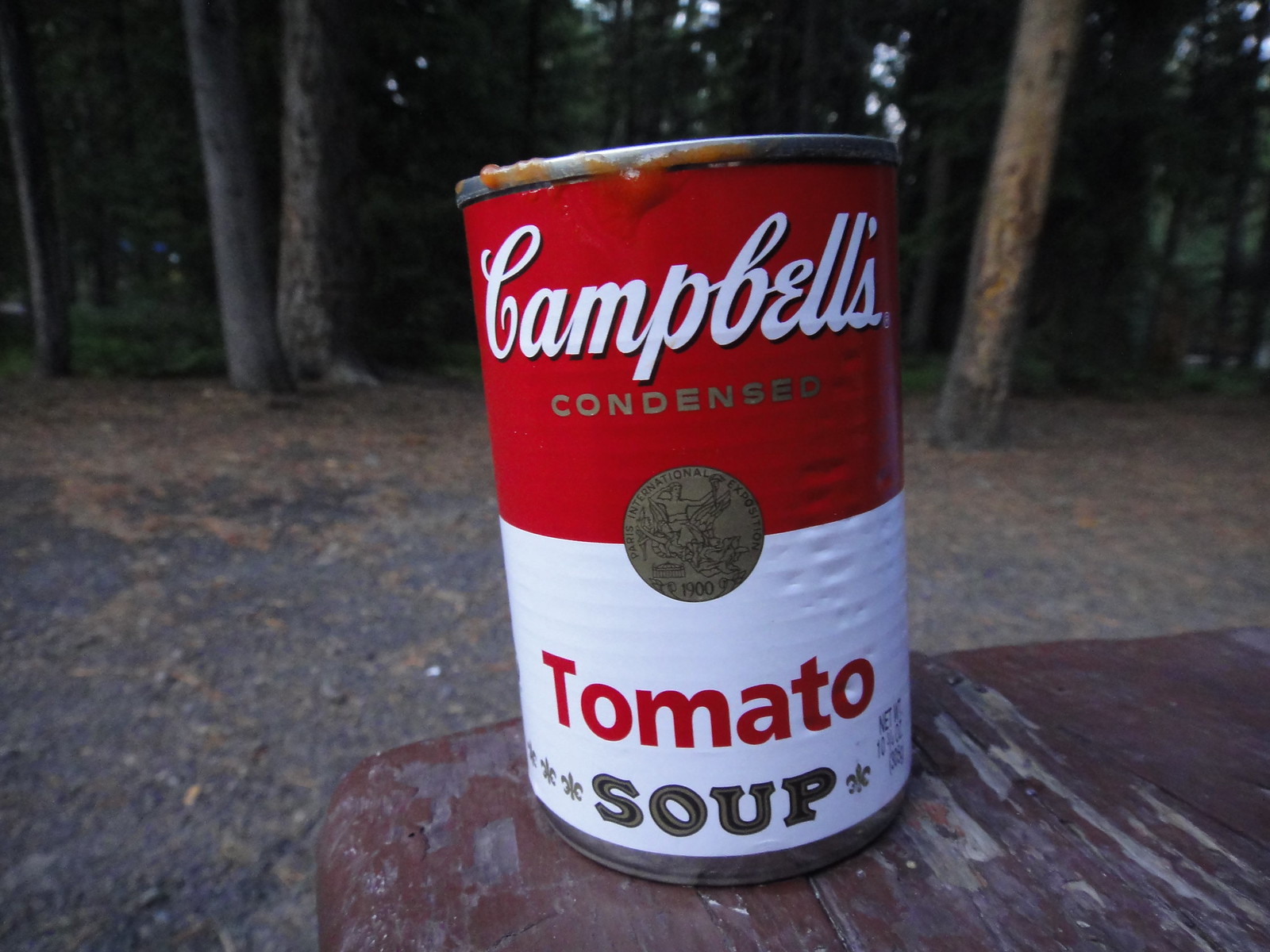This photograph features a can of Campbell's Condensed Tomato Soup prominently displayed outdoors. The can adheres to the classic design with a red upper half emblazoned with "Campbell's" in white, and a white lower half featuring "Condensed" in gold. Below that, a circular medallion labels the "Paris International Exposition 1900" with a logo, followed by "Tomato" in red and "Soup" in silver with star accents. The can appears to have been opened, as there are splotches of red tomato soup around the gray metal rim at the top. It rests on a rough, weathered wooden table that has chipped brown paint revealing white patches underneath. The background reveals a natural setting with gray and brown flooring, possibly gravel, and blurred tree trunks and foliage, with a hint of light blue sky peeking through the leaves.